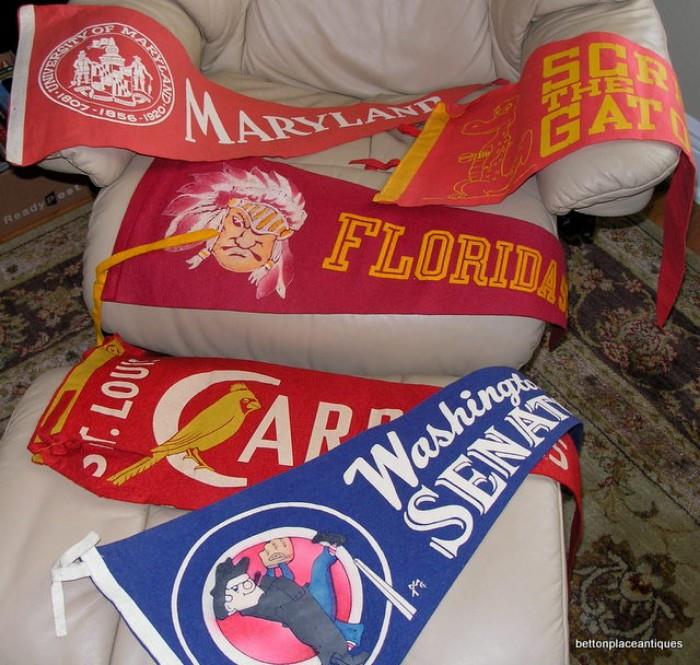This image captures a collection of vintage college and sports pennants artfully draped across a beige leather recliner and its matching ottoman, set against a floral-patterned carpet. Prominently featured are banners for the University of Maryland, with a bold red and white design, and another partially visible red and gold banner suggesting a school with “Gator” in its name. Below these, a Florida State University pennant displays a classic Seminole logo in red and gold. On the Ottoman, there are two more pennants: a red St. Louis Cardinals banner with a cardinal perched on the "C," and a blue Washington Senators pennant featuring a cartoon senator poised to pitch a baseball. Additional details include a small, white, all-lowercase watermark reading "Betten Place Antiques" at the bottom right, likely indicating the seller. The vintage nature of the pennants and the composition of the photograph suggest it was intended for listing on a secondhand marketplace.